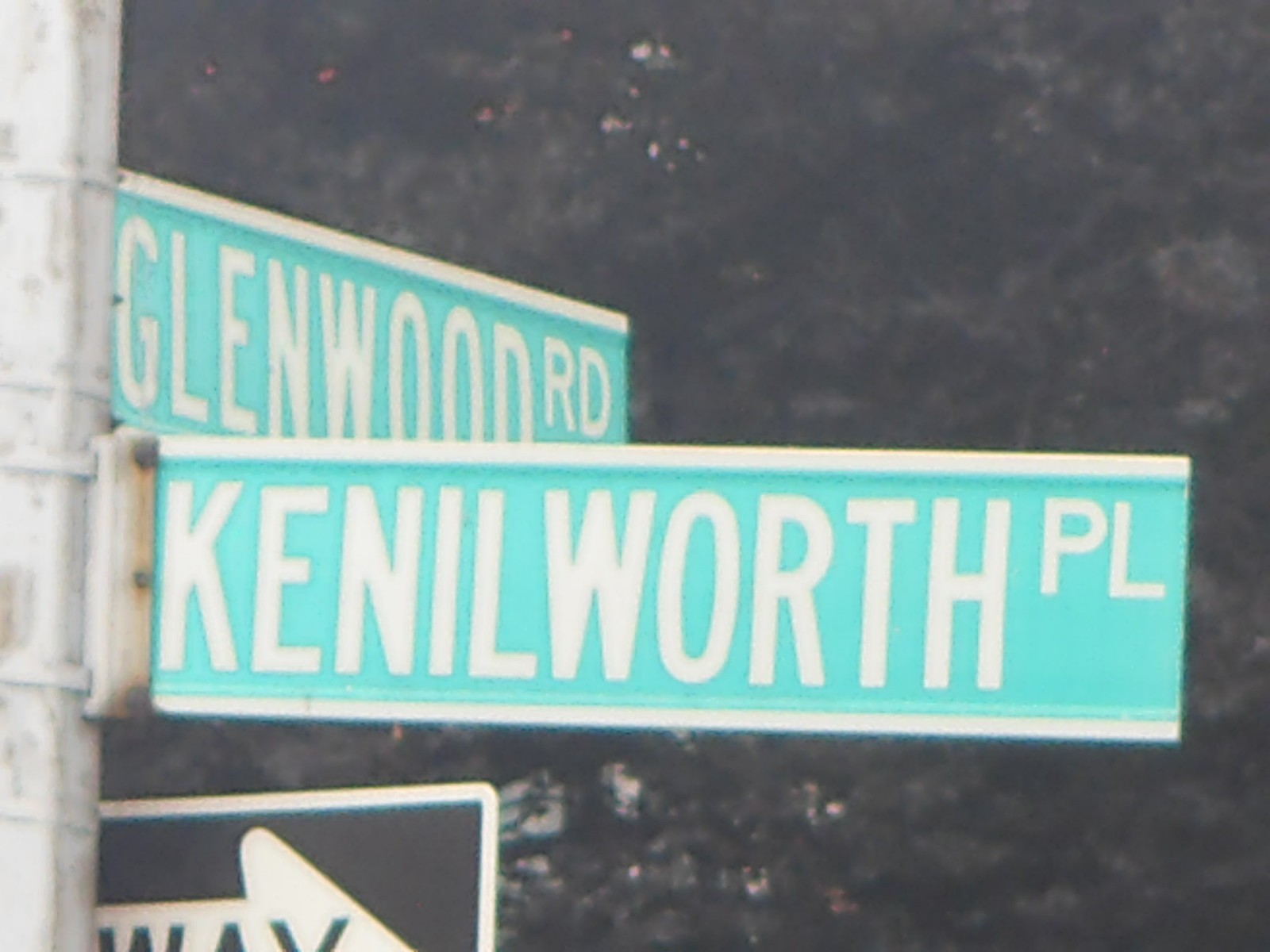This close-up photograph captures a cluster of street signs affixed to a cylindrical gray metal pole positioned on the left side of the image. The central sign dominates the composition with its green background, white borders, and bold white lettering that reads "Kenilworth Place." Perched perpendicularly above it is an identical green and white sign declaring "Glenwood Road." In the lower left corner of the photo, partially cropped, is a black and white one-way sign, revealing only the upper right portion marked by the word "WAY" and a right-pointing arrow. The scene is backdropped by a dense curtain of green foliage, likely from an abundance of trees, adding a lush, natural element to the urban setting. Despite the clarity in details, the image has a noticeable haze, rendering it slightly out of focus.